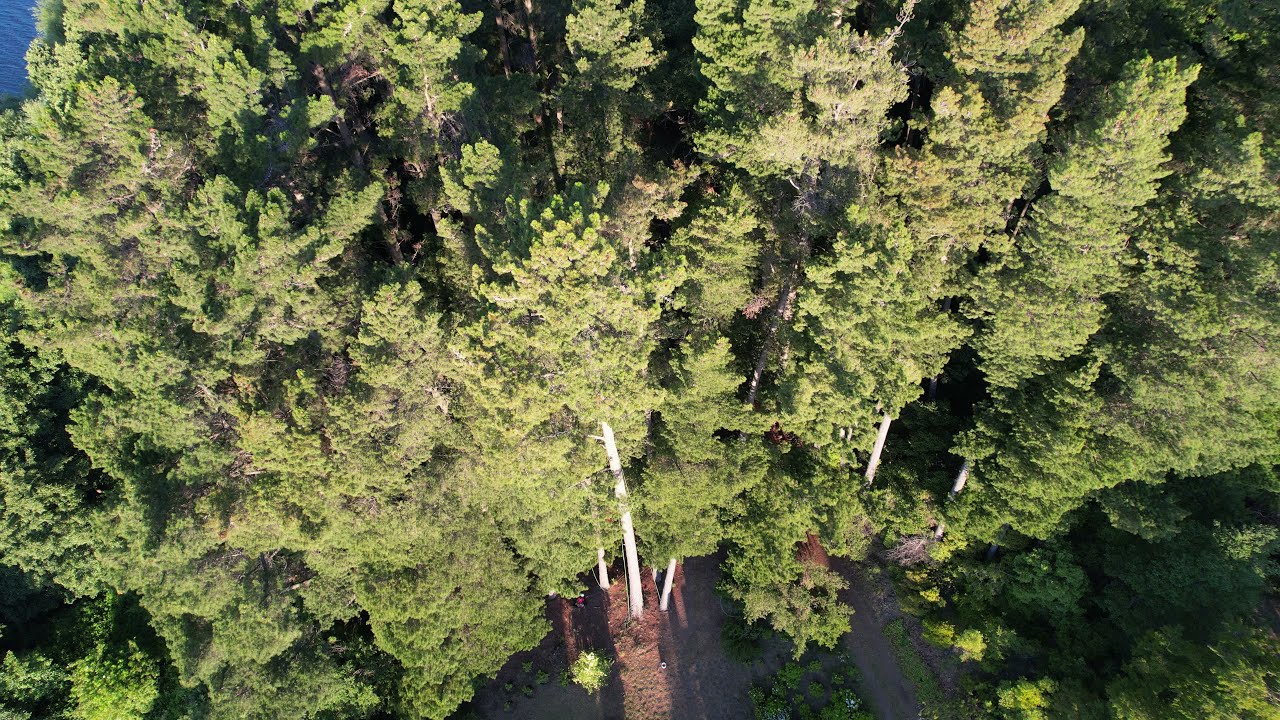The aerial shot captures a dense, sunlit forest with a multitude of light green trees stretching vertically, their slender white trunks accentuated by the sunlight, casting soft shadows on the lower right side. The forest scene is interspersed with a small brown patch of dirt in the center, possibly indicating a narrow dirt road or clearing. In the upper left corner, a glimpse of pristine blue water suggests the presence of a small lake or pond. The leaves are vibrant and lush, covering most of the scene except for the small exposed ground area and the tiny corner of water. This richly textured natural landscape, with its varied shades of green and scattered visual elements, reflects the tranquility and vastness of an uninterrupted forest viewed from above.